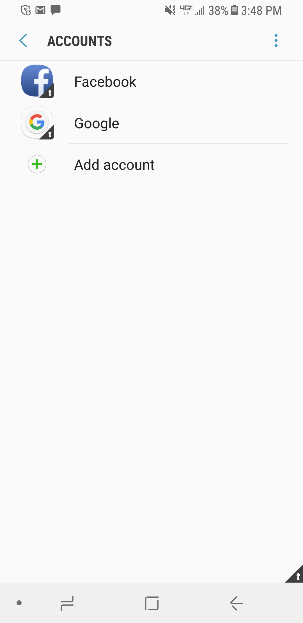This detailed image caption highlights the status of a smartphone displaying the "Accounts" page. The screenshot appears to be from an Android device, given the interface design. The battery level shows 38% remaining. Prominently featured is the "Accounts" section, showcasing two accounts: Facebook and Google. The Facebook account is represented with its iconic white 'F' on a blue background, accompanied by a small indicator labeled "1" in the bottom right corner. Similarly, the Google account is identified with a multi-colored 'G' on a white background, also marked with "1" in the bottom right corner. Additionally, there's a green arrow symbol suggesting the option to add more accounts. This page allows users to manage their integrated accounts on the device.